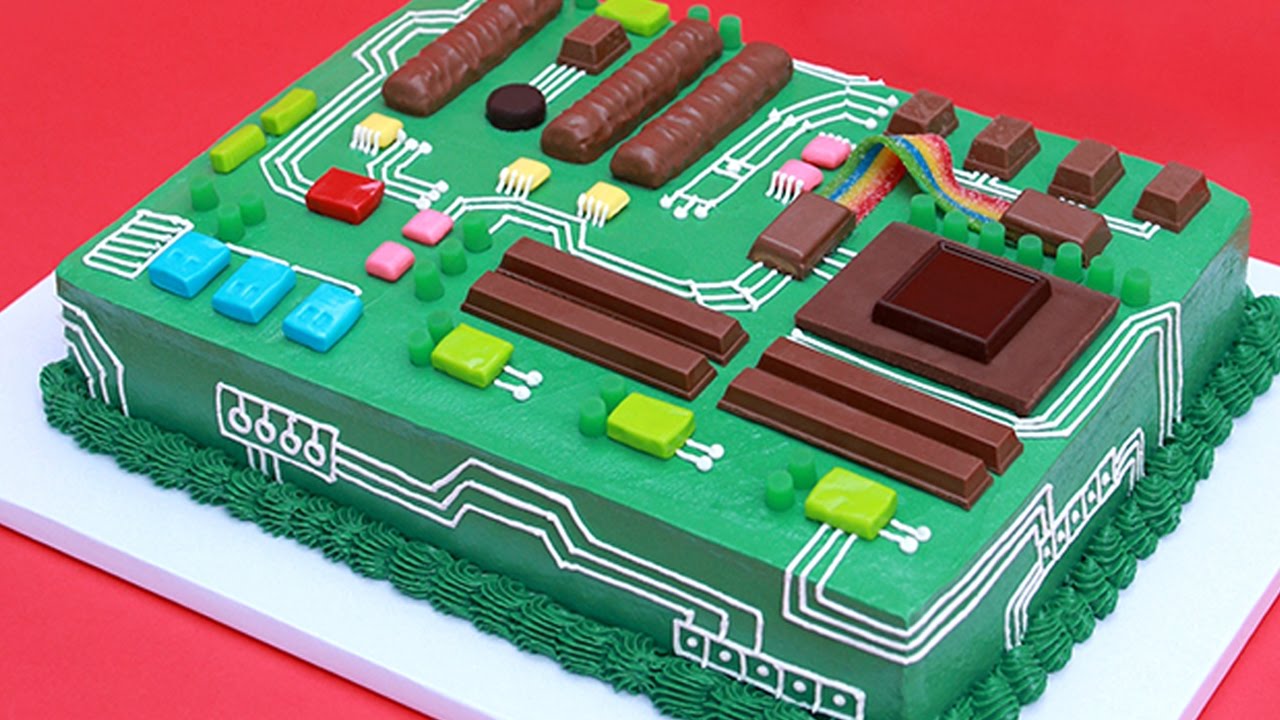The image features a rectangular, green-frosted cake designed to mimic a printed circuit board, with intricate details enhancing its lifelike appearance. The cake rests on a white rectangular platform against a solid red background. The green frosting serves as the base color, while white frosting lines depict the intricate circuits typical of a motherboard, extending in parallel, diagonal, and horizontal patterns. The edges of the cake are adorned with ribbed, bag-pipe style green frosting. Various candies and chocolates, including Twix bars, Kit-Kat bars, chiclet gums, Starburst-like candies, and smaller chocolates, are meticulously placed to represent integrated circuits, microprocessors, and other electronic components. Notably, there is a ribbon cable crafted from licorice, adding a clever touch to the design. Prominent patterns include rows of rectangle and square candies, connected by white frosting lines, simulating the wiring. This detailed, edible creation might be a centerpiece for a computer repair enthusiast's birthday celebration.